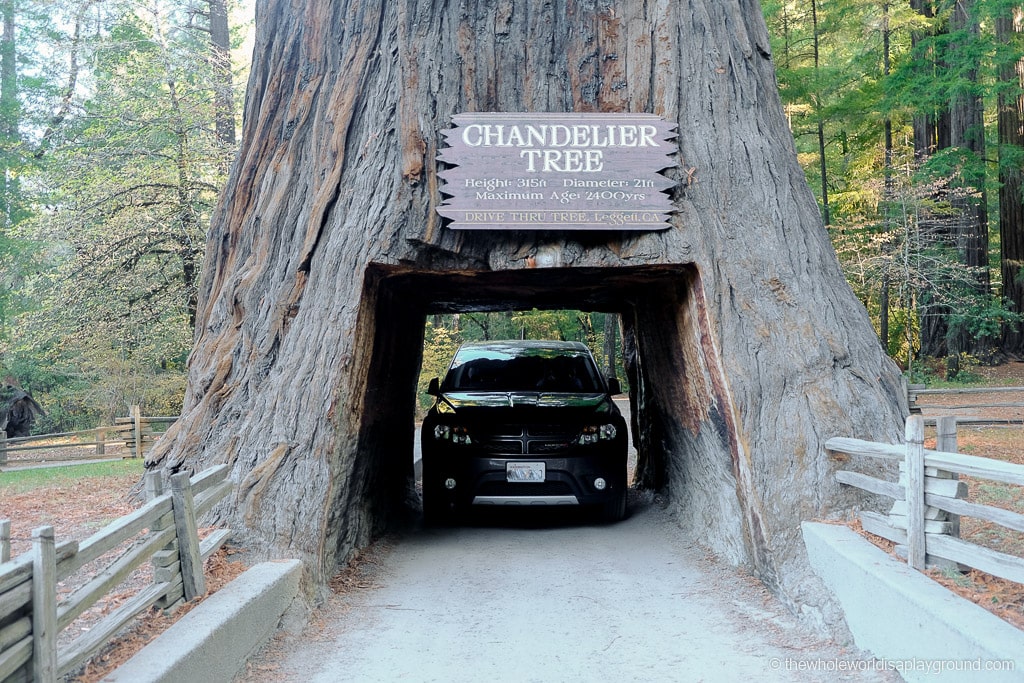In this picture taken outside in a forested area, a massive tree known as the Chandelier Tree stands prominently. Towering at 315 feet, with a 21-foot diameter, this ancient tree, estimated to be 2,400 years old, has a remarkable feature: a carved-out tunnel at its base that allows vehicles to drive through. Visible through this tunnel is a large black car, which appears to be either a larger sedan or a small SUV. Above the tunnel, a light brown wooden sign with jagged edges displays the tree's name in capital letters, "Chandelier Tree," along with statistics about its height, diameter, and age. Additional text on the sign reads "Drive Through Tree, LEGGETT, CALIFORNIA," indicating the location. The background shows a sparse arrangement of trees through which sky can be seen, a wooden fence along the side and front, and a gray cement road leading up to and through the tree. The ground features brown leaves and green grass, adding to the natural setting.